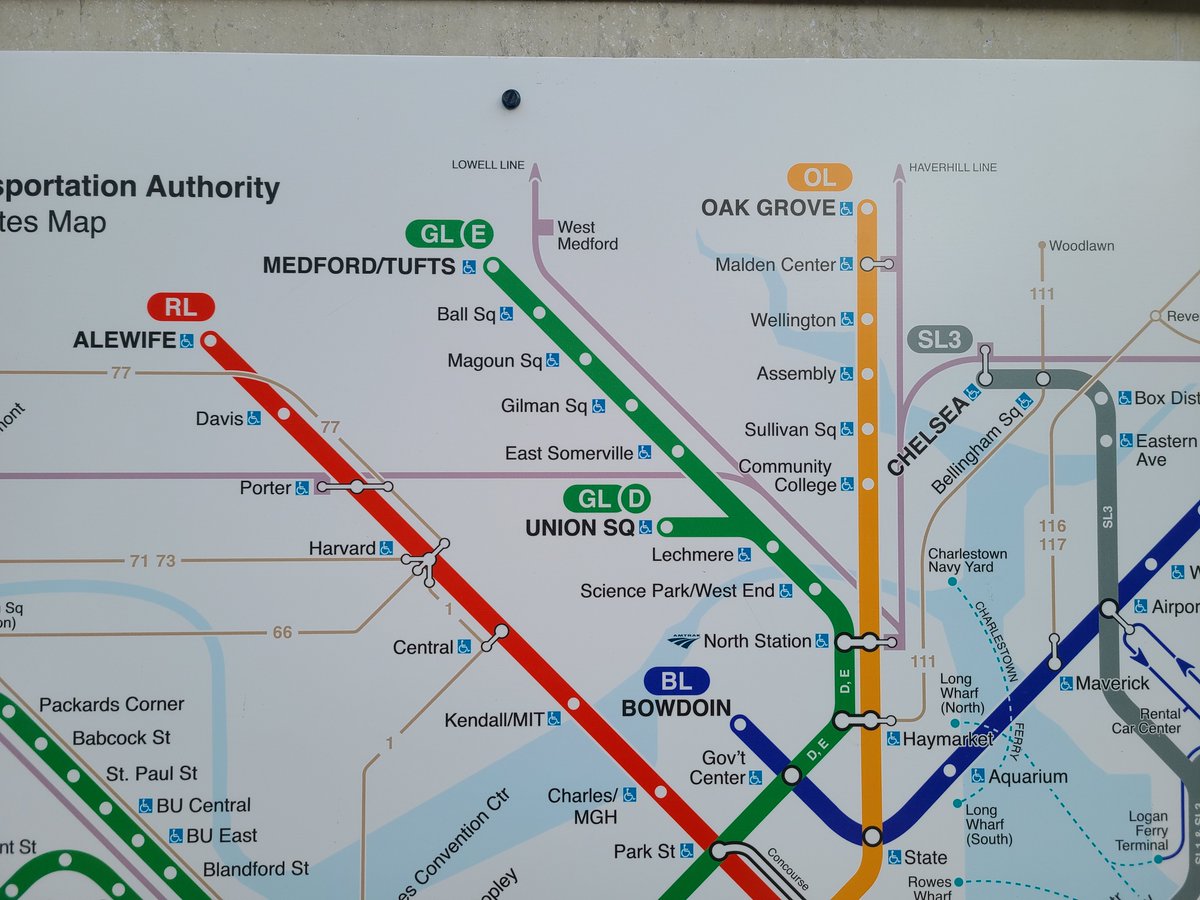This is a color photograph of a detailed map pinned to a wall, likely depicting various railway or subway routes of a transportation system, possibly in Boston, given the references to local landmarks and universities such as MIT and Harvard. The white sheet features numerous multi-colored lines representing different routes: a red line to the left, a green line in the middle, a yellow and blue line to the right, and a gray line further right. Each line is marked with white circles indicating stops at locations including Union Square, Science Park, North Station, Bowdoin, Chelsea, Bellingham Square, Sullivan Square, Aquarium, Community College, Attaway, Davis, Porter, Harvard, Central, and Kendall. The top section of the paper includes partially visible text suggesting it's a notice from the transportation authority, although part of the text is cut off, only showing "Portation Authority." The map appears to be situated indoors, potentially photographed with natural light, and shows a countertop edge at the very top.